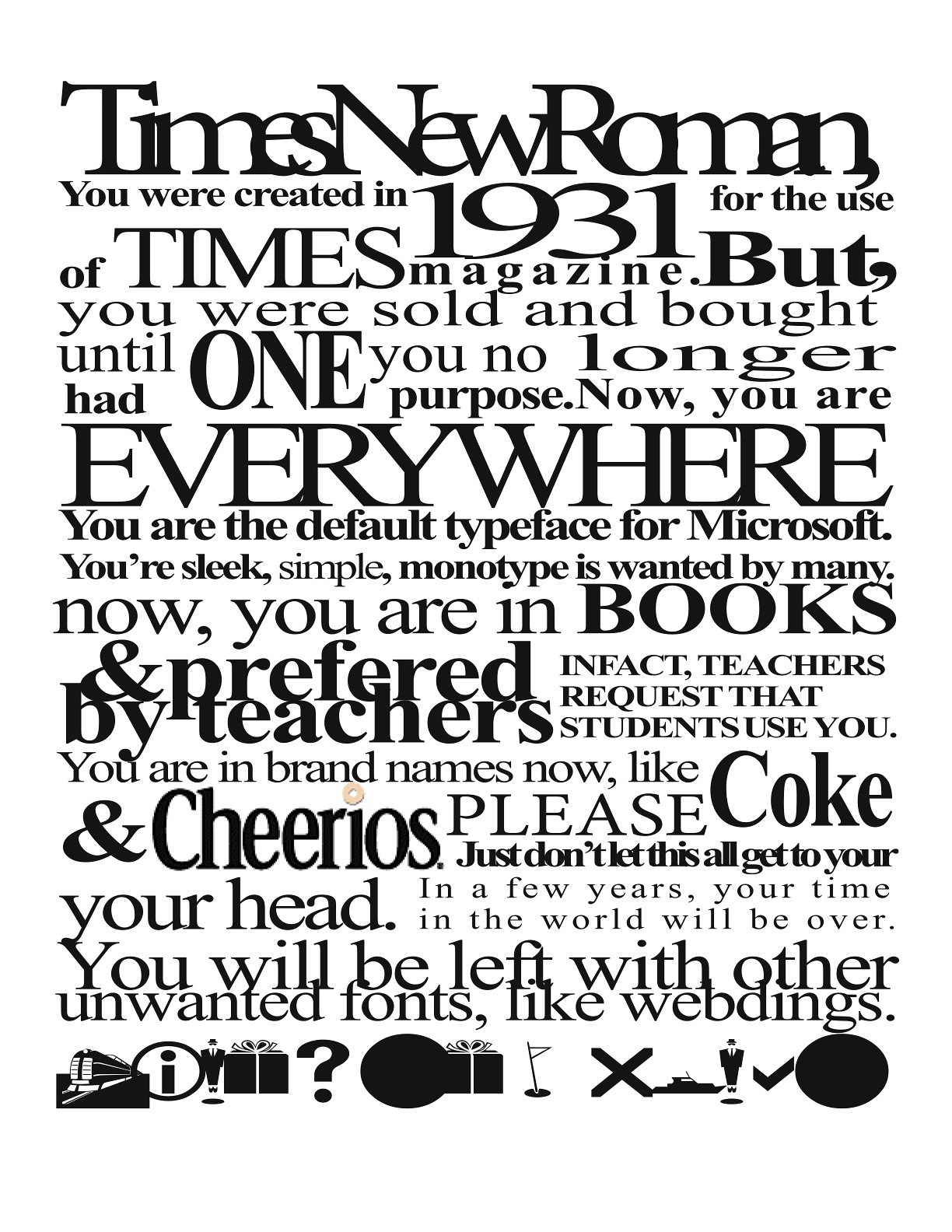This black-and-white portrait-oriented image is a detailed study in typography, featuring a rich commentary on the typeface Times New Roman. Set against a plain white background without borders, the central text starts in the upper left corner, narrating the history of the typeface: "Times New Roman, you were created in 1931 for the use of Times Magazine, but you were sold and bought until you no longer had one purpose. Now you are everywhere." The text continues, discussing Times New Roman's ubiquity as the default typeface for Microsoft, its sleek and simple monotype design, and its widespread usage in books and brand names like Coke and Cheerios. The commentary cautions the typeface not to become overconfident, as it will eventually become obsolete like other unwanted fonts such as Webdings.

The text varies in size, some in bold and large print, and others in much smaller fonts, creating a dynamic visual contrast. At the bottom of the image is a row of black-and-white icons, including a train, a person, a question mark, a golf flag, a present, a circle, and several other symbols. The style is a combination of fun and informative graphic design, effectively using typography to tell the story of Times New Roman through different fonts and styles, culminating in a compact yet visually engaging layout.